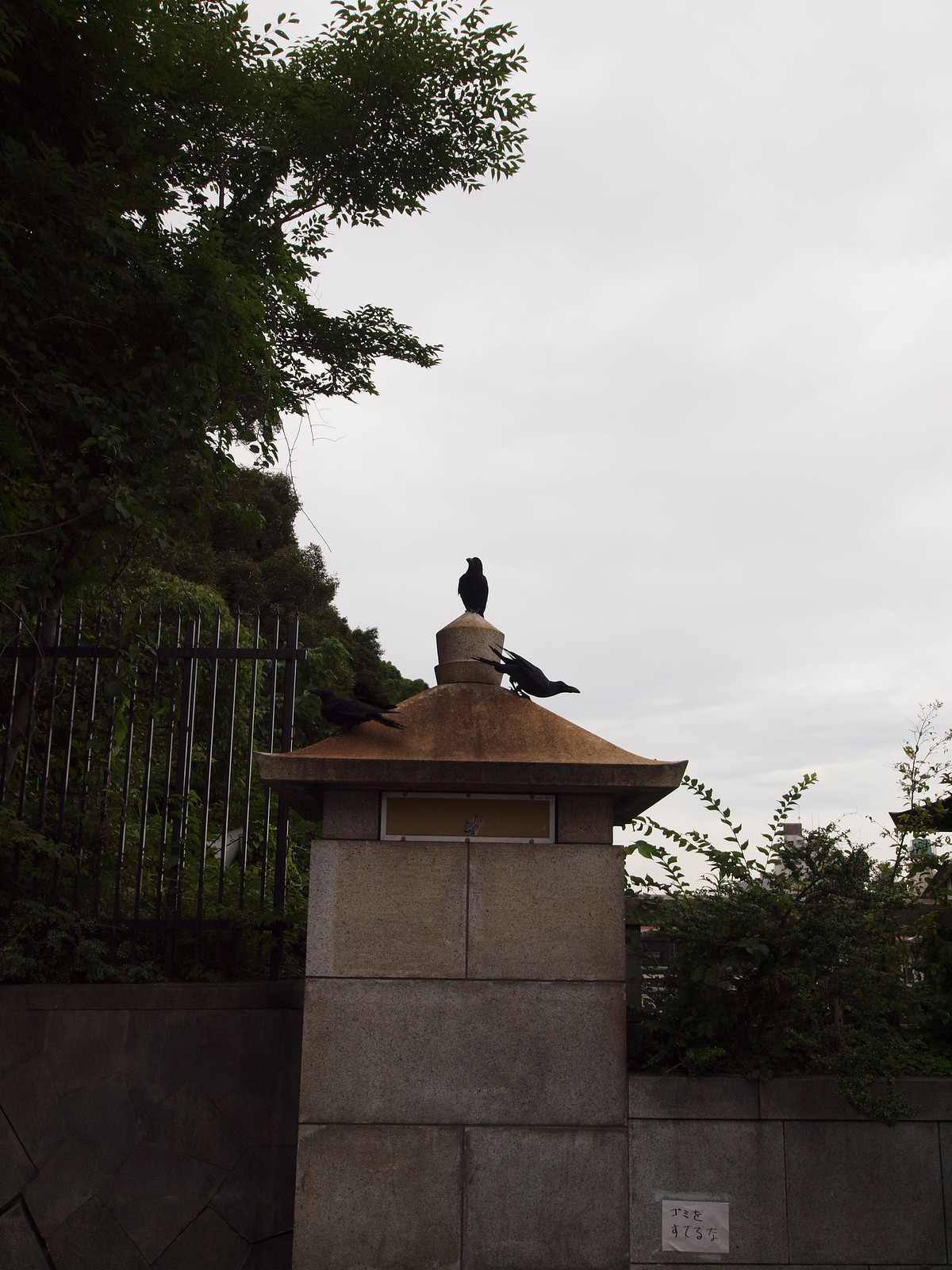The image depicts an outdoor scene under a cloudy, gloomy sky. Dominating the left side of the picture, a cement stone wall, featuring a wrought iron gate with ornate detailing on top, tapers down with the landscape. The wall includes a large pillar crowned with a bronze cap, from which emerge two black birds, likely crows, one poised on the tip and the other with wings spread, ready to take flight. Adjacent to this, a lower cement wall bears an unreadable sign and is adorned with greenery. In the background, trees populate a slight hill, contributing to the scenic depth and varied elevation throughout the composition.